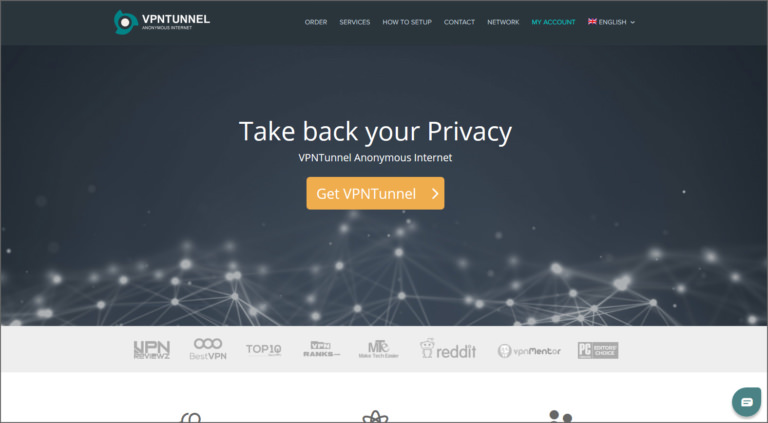The homepage of the VPN Tunnel website features a sleek black background with contrasting white text, creating a modern and straightforward design. In the upper left-hand corner, a logo prominently displays the name "VPN Tunnel." To the right, a navigation menu lists several options in white text: "Order," "Services," "How to Set Up," "Contact," and "Network." Additionally, "My Account" appears in blue text, and there is a drop-down menu for selecting the website language, currently showing "English" with a down arrow.

Centered beneath the navigation menu, bold white text declares "Take Back Your Privacy." Directly below this, the phrase "VPN Tunnel - Anonymous Internet" reiterates the website's purpose, followed by a prominent yellow button with white text that reads "Get VPN Tunnel," indicating a clickable call to action.

At the bottom of the page, there are links to various endorsements from well-known entities: VPN, Best VPN, Top 10, VPN Ranks, MTE, Reddit, VPN Mentor, and PC Editor's Choice. Completing the page, an icon for a chat dialogue box sits discreetly in the bottom right-hand corner, offering users immediate assistance.